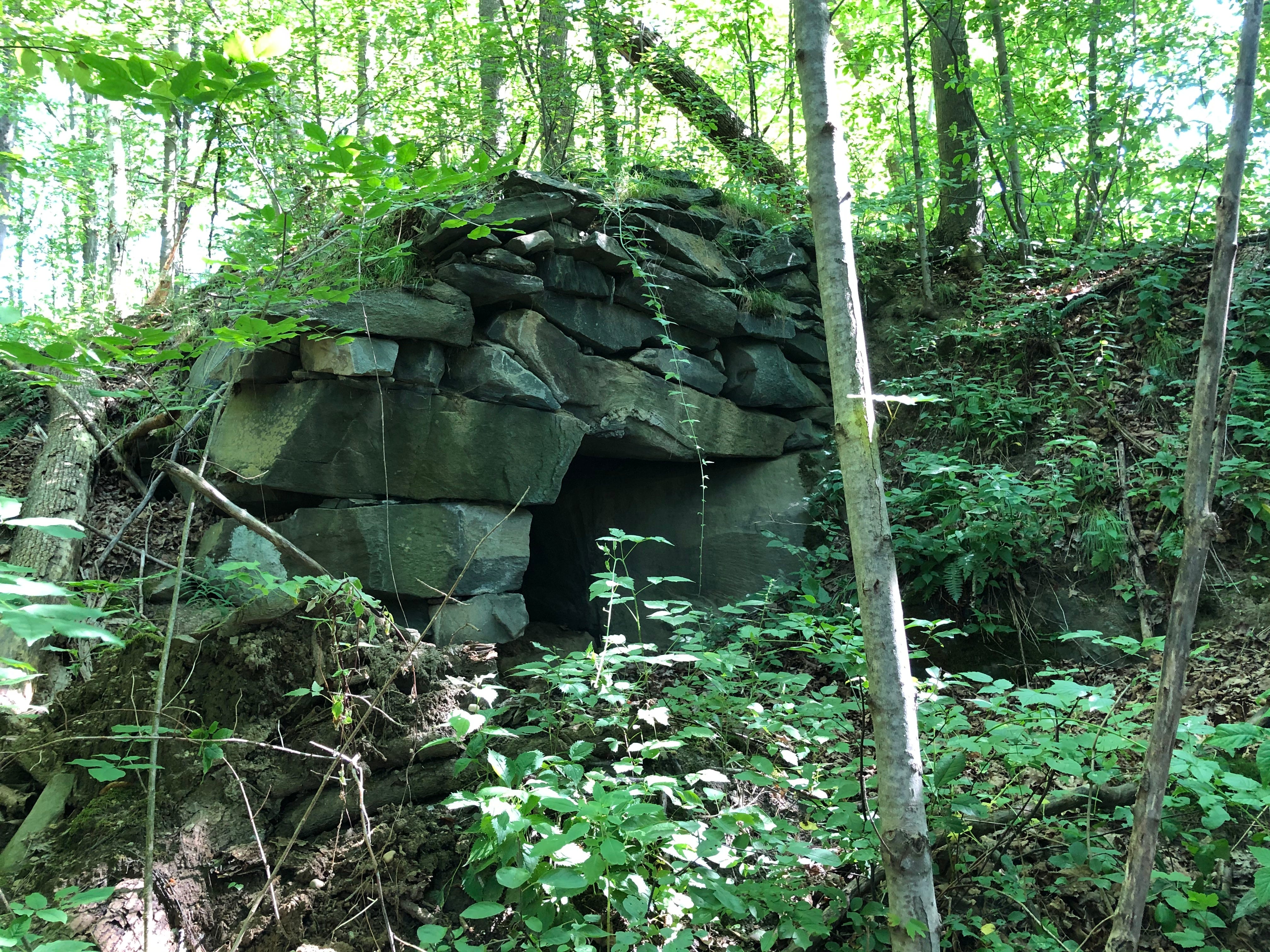In this landscape-style, color photograph, a serene forest teeming with green vegetation surrounds an intriguing, man-made stone structure that resembles the entrance to an ancient cave. The forest is dense with tall, thin trees that could be bamboo, their leafy branches forming a verdant canopy both in the foreground and the background. At the heart of this scene, large, roughly-hewn gray stones meticulously stacked without mortar create an arch that serves as the entrance to the mysterious structure. The entrance, which looks almost like a crafted doorway, reveals a dark and obscure opening inside, its interior cloaked in shadow and unknown depths. The outer stones and much of the structure are blanketed in dirt and plant life, emphasizing the age and natural integration of this enigmatic formation with its woodland surroundings.